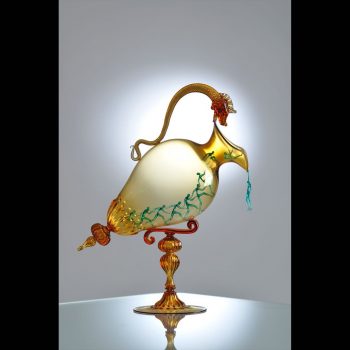This highly detailed photograph captures an ornate, artistic glass pitcher prominently displayed on a reflective surface, illuminated by bright lighting that highlights its vivid colors. The background features a gray setting framed by vertical black bars on either side. The pitcher itself has an orange, bulbous base that tapers into a uniquely designed yellow body, which is angled rather than vertical. A striking dragon or snake handle—with an orange body and a red, somewhat serious-looking head—curves majestically from the base to the top of the pitcher, its mouth poised as if about to close on the spout. Adding to the artistic impression, there's a blue, glass-like liquid seemingly trickling out of the pitcher, mimicking a realistic flow of water. The overall composition, set against a reflective surface, creates an intriguing interplay of light and color, making the entire piece a captivating work of glass art.